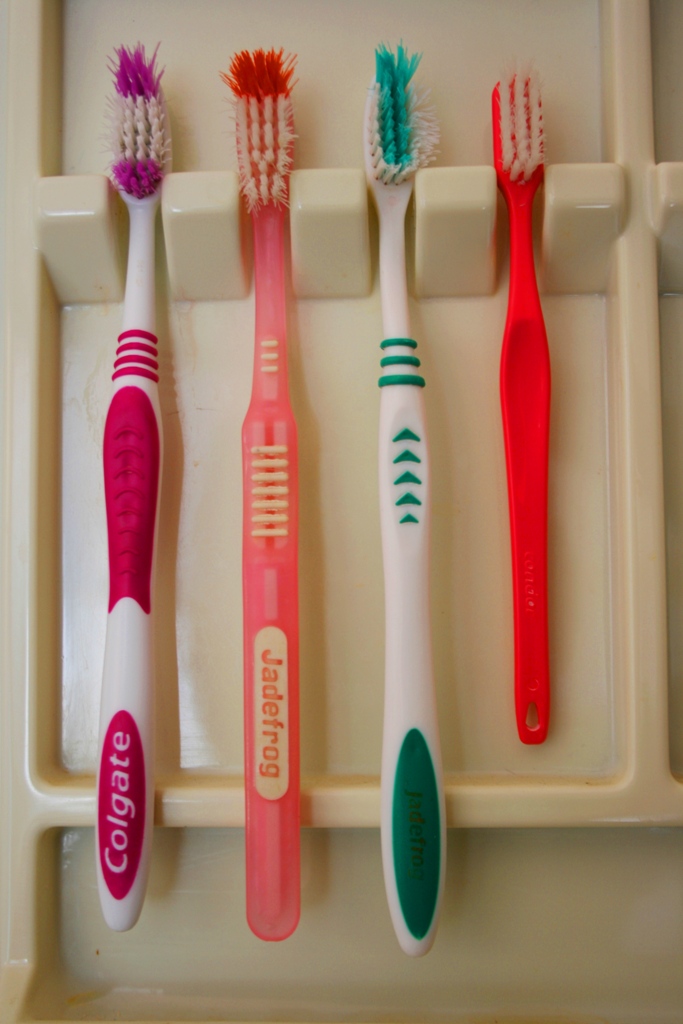The photograph features a cream-colored toothbrush holder, either mounted on a wall or built into a cabinet, with four toothbrushes arranged vertically side by side in designated niches. All four toothbrushes exhibit signs of regular use, with splayed bristles indicative of consistent wear over several months. The first toothbrush on the left is predominantly white with pinkish-red accents and "Colgate" inscribed at the bottom. The second toothbrush is hot pink with white accents, branded as "Jadafrog." The third toothbrush is white with dark green accents, lacking a visible brand name. The final toothbrush is a bold pink, child-sized with comparatively less wear, featuring white bristles. The holder itself is plastic, with individual slots keeping the toothbrushes neatly in place.